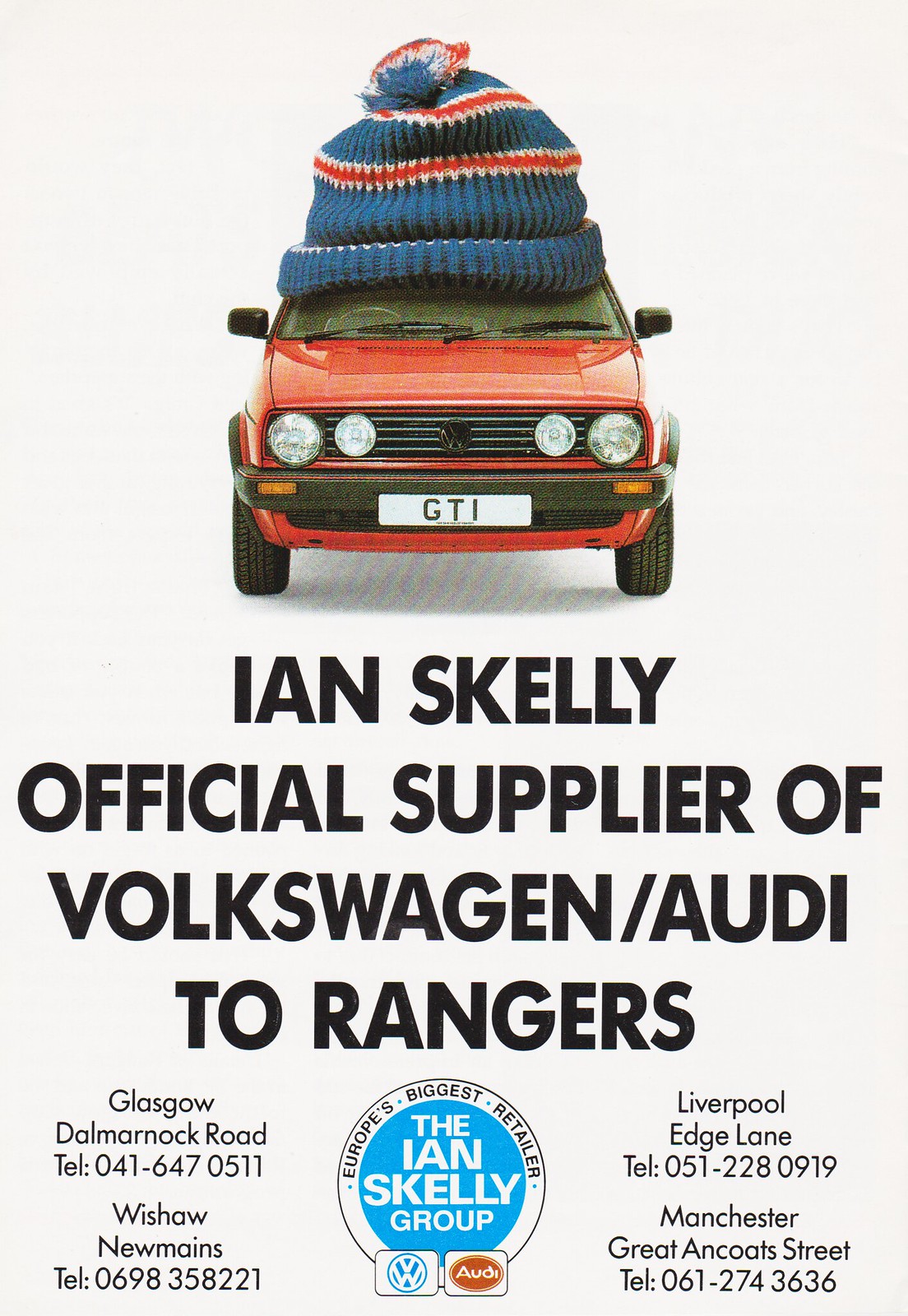The image is an advertisement featuring the front view of an orange hatchback car adorned with four headlights and two visible rearview mirrors. A wool ski hat, characterized by its blue and orange stripes and topped with a fuzzy pom-pom, sits whimsically on the car’s roof. The bumper bears the "GTI" insignia, subtly indicating the car model. Beneath the car, text prominently states "Ian Skelly, official supplier of Volkswagen/Audi to Rangers," accompanied by various contact details including locations and telephone numbers: Glasgow-Dalmarnock Road (041-647-0511), Wishaw New Mainz (0698-358-221), Liverpool Edge Lane (051-228-0919), and Manchester Great Ancote Street (061-274-3636). The advertisement also showcases the logos of Volkswagen and Audi alongside the Ian Skelly Group emblem, underscoring its European retail dominance.